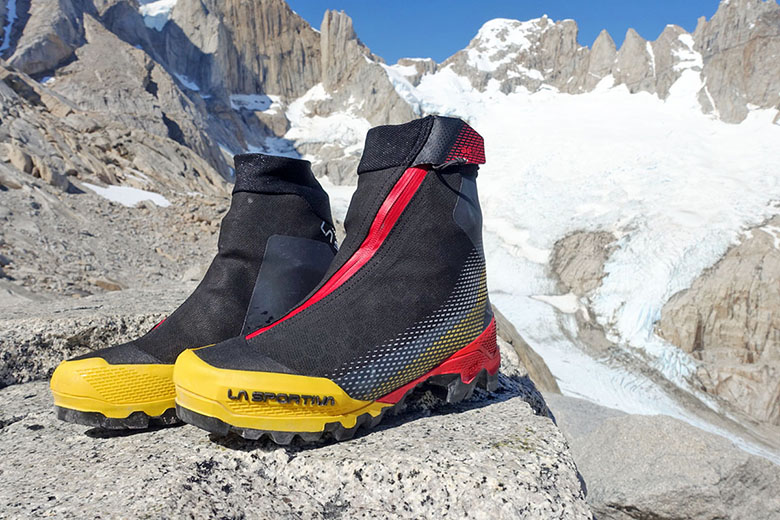This outdoor photograph captures a pair of distinct hiking boots prominently displayed in the foreground. These boots are predominantly black with a scattering of white dots and feature yellow toes and a red heel, accompanied by a diagonal red zipper stripe. The outer side of the left boot is inscribed with the brand name "La Sportiva." The boots rest on a gray, speckled rock formation, enhancing their rugged appearance. In the background, a panoramic view of majestic, snow-covered gray mountains stretches across the scene, with a pristine blue sky overhead, unmarred by clouds. The bright sunlight illuminates the landscape, emphasizing the contrast between the white snow and the rocky terrain, thereby creating a vivid and picturesque setting.